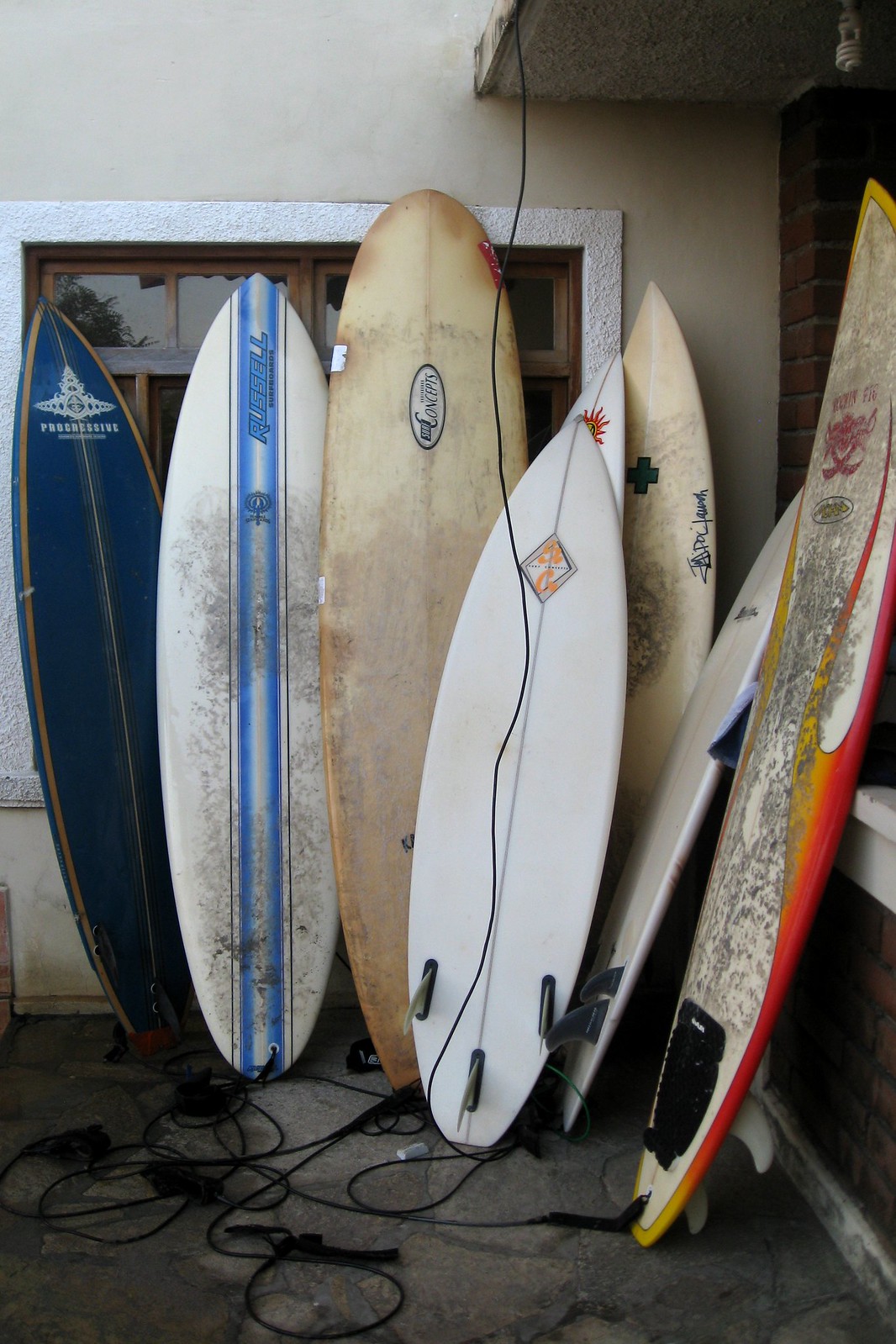This photograph captures a collection of eight surfboards leaning against a corner wall, combining a white plaster and brick exterior. The setting appears to be outdoors, possibly adjacent to a house or a storage area. 

The wall features a brown wooden-framed window bordered by a white stucco extrusion, below which the surfboards rest on a cement floor with visible patches of brick and scattered black leashes. Above, a wire dangles from a second-story balcony, ending in a curly, soft-serve shaped fluorescent bulb.

From left to right, the surfboards display a variety of colors, conditions, and designs:

1. A navy blue surfboard with yellow trim, marked "Progressive" alongside an intricate logo.
2. A white surfboard with a blue vertical stripe in the middle, labeled "Russell."
3. An aged, beige surfboard bearing the "Concepts" logo within an oval. This board appears patched and worn.
4. A smaller white surfboard with three fins (tri-fin setup), showing signs of mildew and dirt.
5. Another slightly obscured white surfboard adorned with a sunburst logo.
6. A creamy tan surfboard, pointy at the tip, featuring a green cross emblem.
7. A second white surfboard with visible fins extending forward.
8. A heavily waxed board covered in dirty black wax, primarily white but accented with red and yellow flame-like stripes.

All the surfboards show varying degrees of wear, with some appearing moldy and others bearing visible dirt, indicative of extensive use or long-term storage. The eclectic mix of shapes and sizes demonstrates an intriguing assortment of surfboards possibly awaiting use or repurposing.